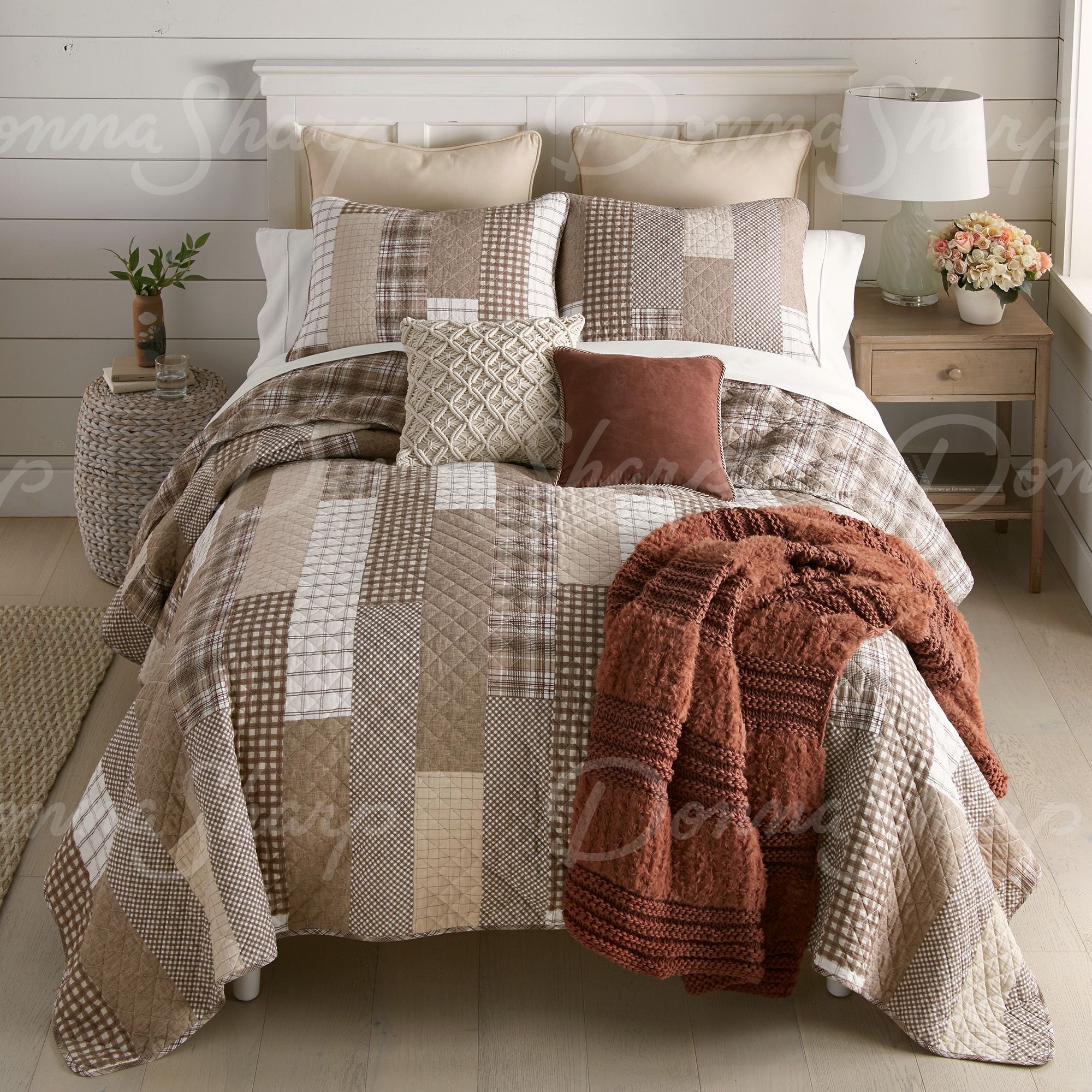The image depicts a stylized bedroom with a hobo-rustic design, featuring a prominent bed with a quilt blanket made of various plaid patterns in soft natural colors such as brown, camel, beige, and reddish-brown. The bed is turned down, displaying a layered setup with multiple throw pillows, including a purple one, white embroidered ones, larger brown plaid ones, and beige ones, alongside the standard pillows. A comforter draped over the foot of the bed adds to the coziness. 

To the right of the bed stands a light brown wooden night table with a white ceramic flower pot housing green, pink, and yellow flowers, next to a lamp with a white shade and a bouquet of flowers. On the left, there's an enclosed wicker basket holding a glass of water and a small potted plant. The room is accented with horizontal wood panel walls painted white, alongside white baseboards and light brown or grayish hardwood or linoleum floors. A rough light brown rug with a diamond grid pattern lies to the left. 

The backdrop includes a white-painted wooden headboard, complementing the rustic yet homely feel. A window on the right side of the room allows sunlight to stream in, illuminating the overall tranquil and cozy ambiance of the bedroom.